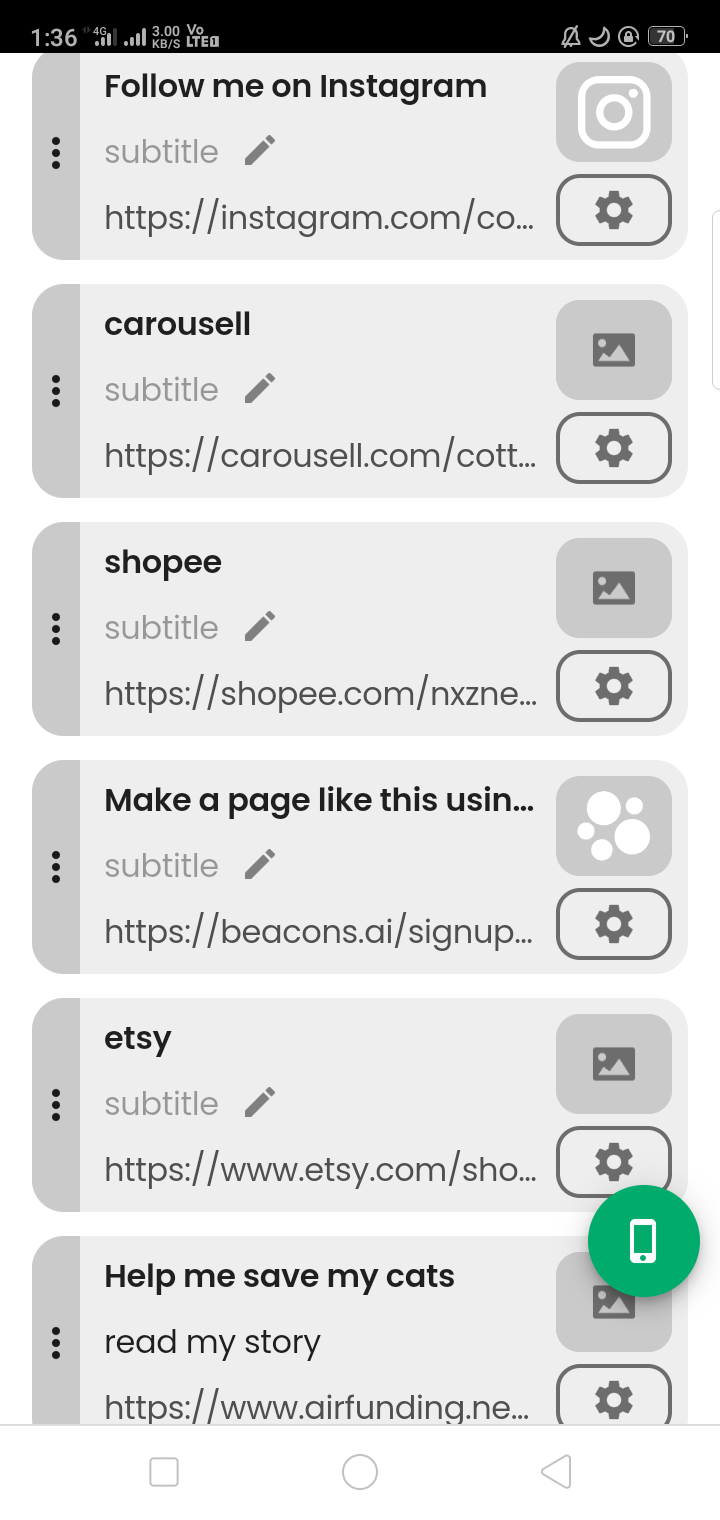The image is a vertically rectangular screenshot of a cell phone screen. At the very top, there is a narrow black horizontal banner displaying the time as 1:36, accompanied by various icons, including a Wi-Fi signal bar. Beneath this banner, there is a vertical list of websites, each enclosed in a horizontally rectangular background.

The first item in the list is labeled "Follow me on Instagram," with an Instagram button and a settings button to its right. The partial web address "https://instagram.com" is visible beneath it.

The second item is titled "Carousell" (spelled with two L's) and includes a picture button along with a settings button to its right.

Following this is an item labeled "Shop e," which has an associated web address of "https://beacons.ai."

Next in the list is "Etsy," but no additional details are provided for this entry.

The final item reads "Help me save my cats," suggesting a personal or charitable appeal, though no further context or details are given.

Each of these items is neatly organized in a list format, making the interface appear user-friendly and navigable.